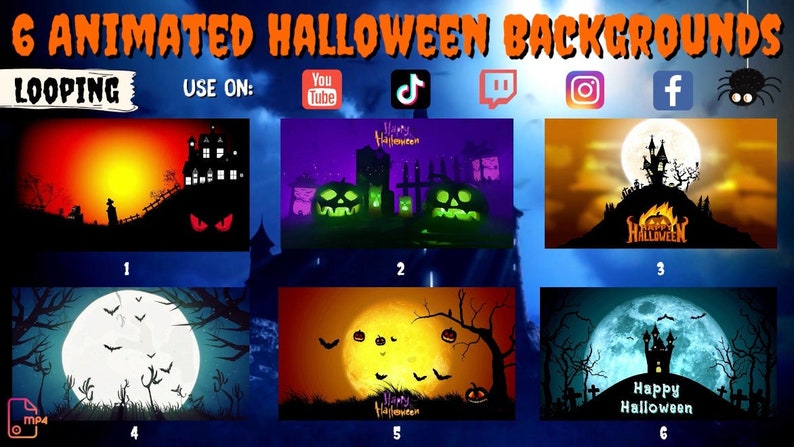The image is a digital screenshot featuring an advertisement for "Six Animated Halloween Backgrounds." The title is prominently displayed at the top in a creepy, orange font reminiscent of classic horror themes, set against a dark backdrop. Beneath the banner, the description "looping Halloween backgrounds" emphasizes that these animated scenes seamlessly repeat in a manner where the transitions are imperceptible.

The display is organized in a 3x2 grid, showcasing thumbnails of the six distinct Halloween-themed animated wallpapers. 

1. The first thumbnail depicts the silhouette of people approaching a haunted house, their dark figures outlined against an eerie, illuminated background.
   
2. The second image presents a nightmarish graveyard filled with green-lit jack-o'-lanterns, shrouded in purple smoke, creating a surreal and spooky atmosphere.
   
3. The third wallpaper illustrates a sinister, Tim Burton-esque house perched atop a hill, silhouetted against a full moon that bathes the scene in a ghostly glow.
   
4. The fourth background offers a close-up view of an enormous full moon bordered by the dark silhouettes of ominous trees.
   
5. The fifth image features another massive moon, this time with an orange hue. In the foreground, a skeletal tree adorned with black jack-o'-lanterns and bats circling in the night sky contribute to its eerie quality.
   
6. The final wallpaper shows a hyper-realistic, gigantic moon behind a creepy, stylized house on a hill. The foreground is lined with skeletal trees and gravestones, enhancing the haunting ambiance.

Each background is designed to evoke a distinct sense of Halloween spookiness, perfect for setting a chilling tone.